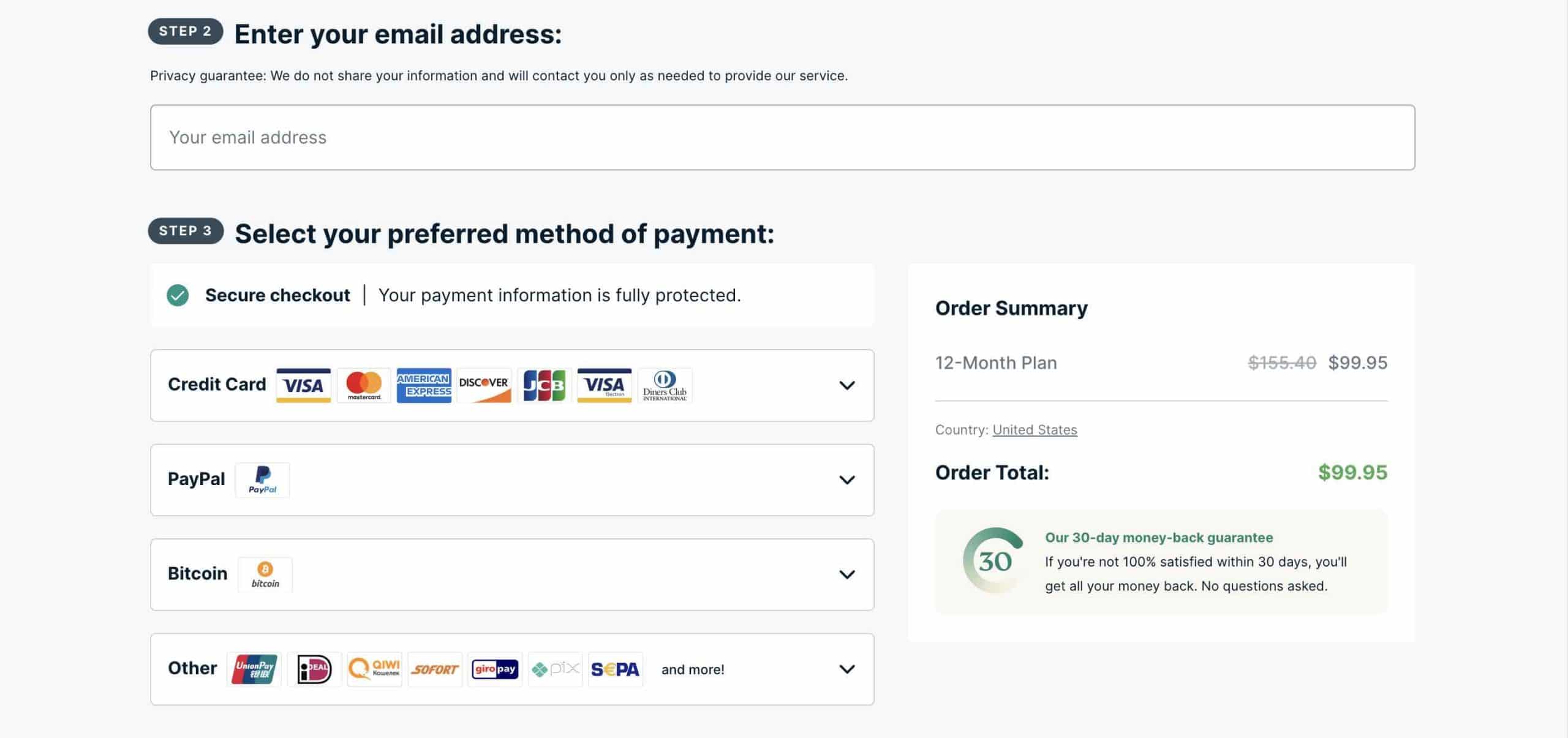**Website Checkout Page Screenshot Description:**

The screenshot depicts a section of a website’s checkout page, displaying key steps and essential information for purchasers.

- **Background and Text:** The background is white with predominantly black text, except for some colored highlights and elements.
  
- **Step Two:** At the top, within a black rectangle, bold white text reads "Step 2." This section prompts users to "Enter your email address." Below this instruction, there is reassurance about the privacy of personal information with the statement: "Privacy guarantee, we do not share your information or contact you only as needed to provide our service." There's an input field spanning the width of the page for users to enter their email address.

- **Step Three:** Following step two, a highlighted section titled "Step 3" guides users to "Select your preferred method of payment." This part emphasizes a "Secure checkout," indicated by a green checkmark symbol with the assurance, "Your payment information is fully protected." A list of payment methods follows, including:
  - Credit Cards: Visa, MasterCard, American Express, Discovery, JCBI
  - PayPal
  - Bitcoin
  - SEPA
  - Google Pay
  - Various other methods which are mentioned but not fully legible.

- **Order Summary Zone:** On the right, an "Order Summary" is provided. It details:
  - **Plan:** A "12-month plan" originally priced at $155.49, now discounted to $99.95.
  - **Country:** United States
  - **Order Total:** Highlighted in green, $99.95

- **Money Back Guarantee:** Beneath the order summary, there is a light green box featuring a "30" rendered in shades from dark green to white, shaped within a nearly complete circle. Accompanying text states: "Our 30-day money back guarantee. If you're not 100% satisfied within 30 days, you’ll get all your money back, no questions asked," in green text.

The page is informative and structured to ensure a secure and transparent buying experience, emphasizing privacy, security, and customer satisfaction guarantees.